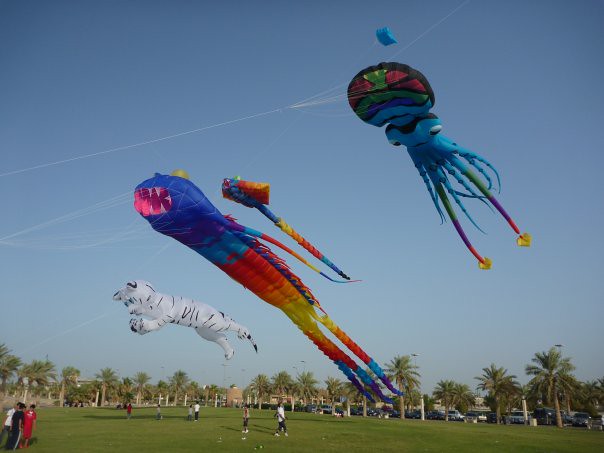On a bright, cloudless day with a few thin wisps of clouds, a group of gigantic kites float majestically in the clear blue sky over a large field. A diverse crowd of people, scattered across the field, interacts with these enormous kites, probably holding their strings. In the background, palm trees and a parking lot full of cars frame the scene, suggesting a festive gathering, possibly a kite flying festival.

From right to left, the largest kite is a vibrant squid with a colorful green and pink carapace, a blue body, and tentacles adorned with shades of green, purple, pink, and yellow. Above this enormous squid, which is larger than several cars put together, there's a small blue box kite. Next to the squid, a smaller but still substantial rainbow-colored kite, with a tail almost as long as a semi-truck, is visible. The kite showcases a gradient of colors from blue and aqua to red, orange, yellow, and back to blue.

Further to the left, there's a sea creature-like kite resembling a lantern fish, characterized by a blue head with a big pink mouth and teeth, and multiple spindly legs in various colors including blue, red, orange, and yellow. Finally, on the far left, a majestic white Siberian tiger kite with striking blue eyes and classic black stripes stretches its paws out as if it's soaring above the crowd. The entire scene, with additional small kites like a blue one in the far background, depicts a vibrant, colorful, and engaging kite flying event against the idyllic sky.